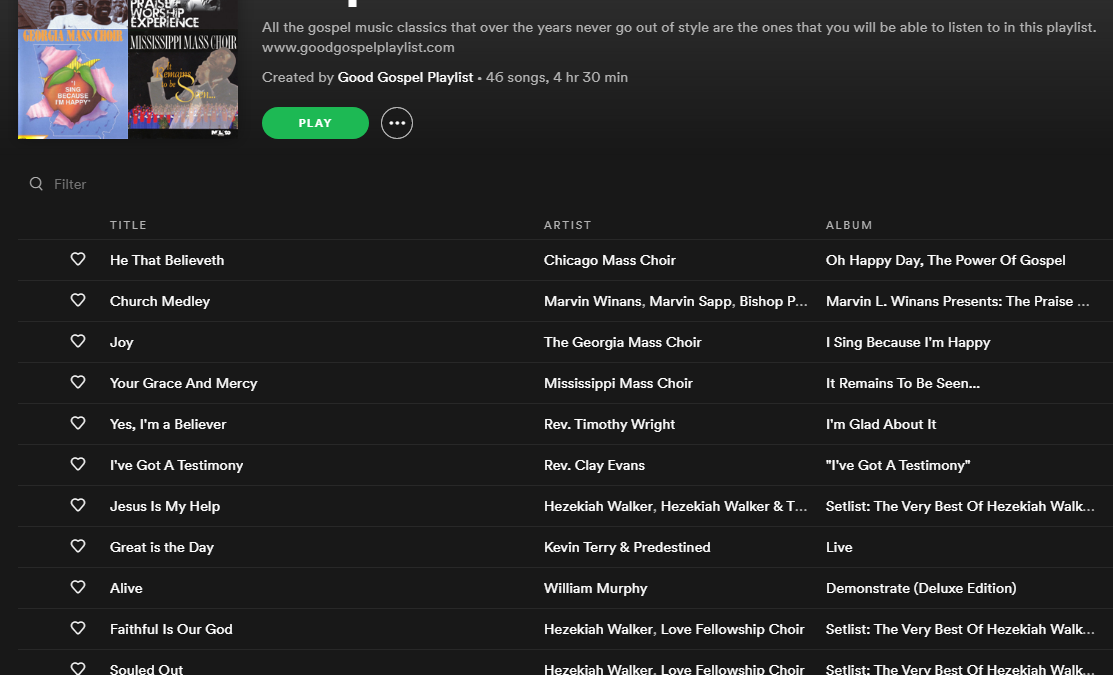The image depicts a music-themed website, specifically a gospel music playlist without a visible title. The website highlights a playlist curated by "Good Gospel Playlist," consisting of 46 songs totaling 4 hours and 30 minutes of playtime. In the upper left corner, there are two album covers; one featuring a large strawberry and the other showing a black man singing. The website's tagline promotes timeless gospel music classics that remain beloved through the years.

The URL displayed on the site is "googlegospelplaylist.com." A prominent green play button is situated at the top, accompanied by a circular icon with three white dots, which likely offers additional options. There is also a filter section with a search icon and a question mark, possibly for sorting and finding specific tracks within the playlist.

The body of the page lists the song titles, artists, and corresponding albums in a structured format. Some of the featured tracks include "He That Delivereth," "Church Melody," "Joy," "Your Grace and Mercy," "Yes I'm a Believer," "I've Got a Testimony," "Jesus is My Help," "Great is the Day," "Alive," "Faithful is Our God," and "Sold Out." The artists mentioned include Chicago Mass Choir, Georgia Mass Choir, Reverend Clay Evans, William Murphy, among others. The albums listed are "Oh Happy Day," "The Power of Gospel," "I Sing Because I'm Happy," "It Remains to be Seen," etc. The entire website is set against a completely black background, providing a stark contrast that makes the text and images stand out.